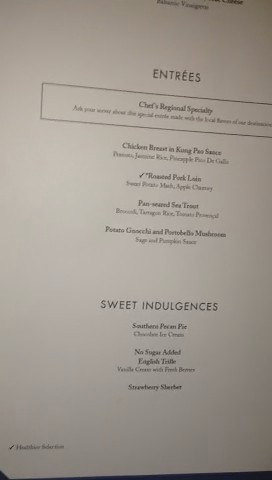Despite its slightly out-of-focus nature, the photograph captures a high-end restaurant menu with a subtle elegance. The top of the menu prominently displays the heading “Entrees,” spelled out as E-N-T-R-E-E-S. Below this, a subtitle reads “Chef's Regional Specialty,” hinting at curated, locale-inspired dishes. Some of the bold entree items discernible through the blur include “Chicken Breast in Kung Pao Sauce,” “Roasted Pork Loin,” and “Pan-Seared Sea Trout.” 

Toward the bottom of the menu, the heading “Sweet Indulgences” introduces the dessert offerings. Among these, “Southern Pecan Pie” and “No Sugar Added English Dessert” are listed, with “Strawberry Sherbet” distinctly highlighted at the bottom. The menu's off-white background and very small, neatly presented text contribute to an air of sophistication and suggest a high-end dining experience.